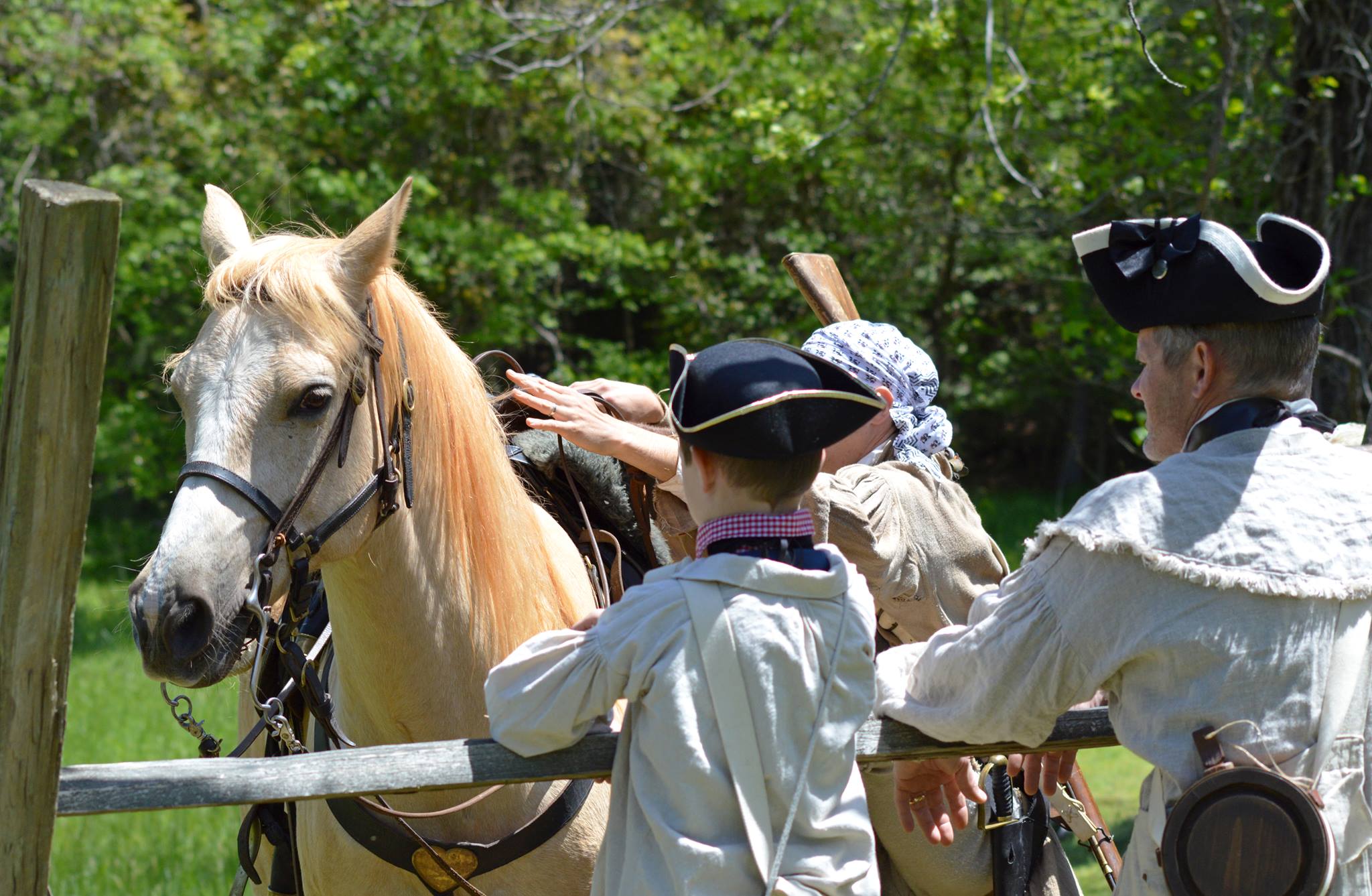The photograph, taken outdoors on a sunny day, depicts a serene green field bordered by a wooden fence, with lush trees in the distance. At the center of the image is a tan-colored horse adorned with a harness around its mouth and a saddle on its back. The horse's mane is notably long and blonde, with hints of red. Near the horse, within the fenced area, stands a man touching the horse, dressed in a tan outfit and a head covering. Outside the fence are two figures, one appearing to be an older man and the other a young boy. Both are wearing traditional white outfits, black hats, and accessories such as a water canteen and possibly a rifle. They are attentively watching the man and the horse, embodying a scene reminiscent of a historical reenactment with Civil War or colonial-era attire. The overall mood is pastoral and timeless, highlighted by the bright sunlight and expansive grassy field.